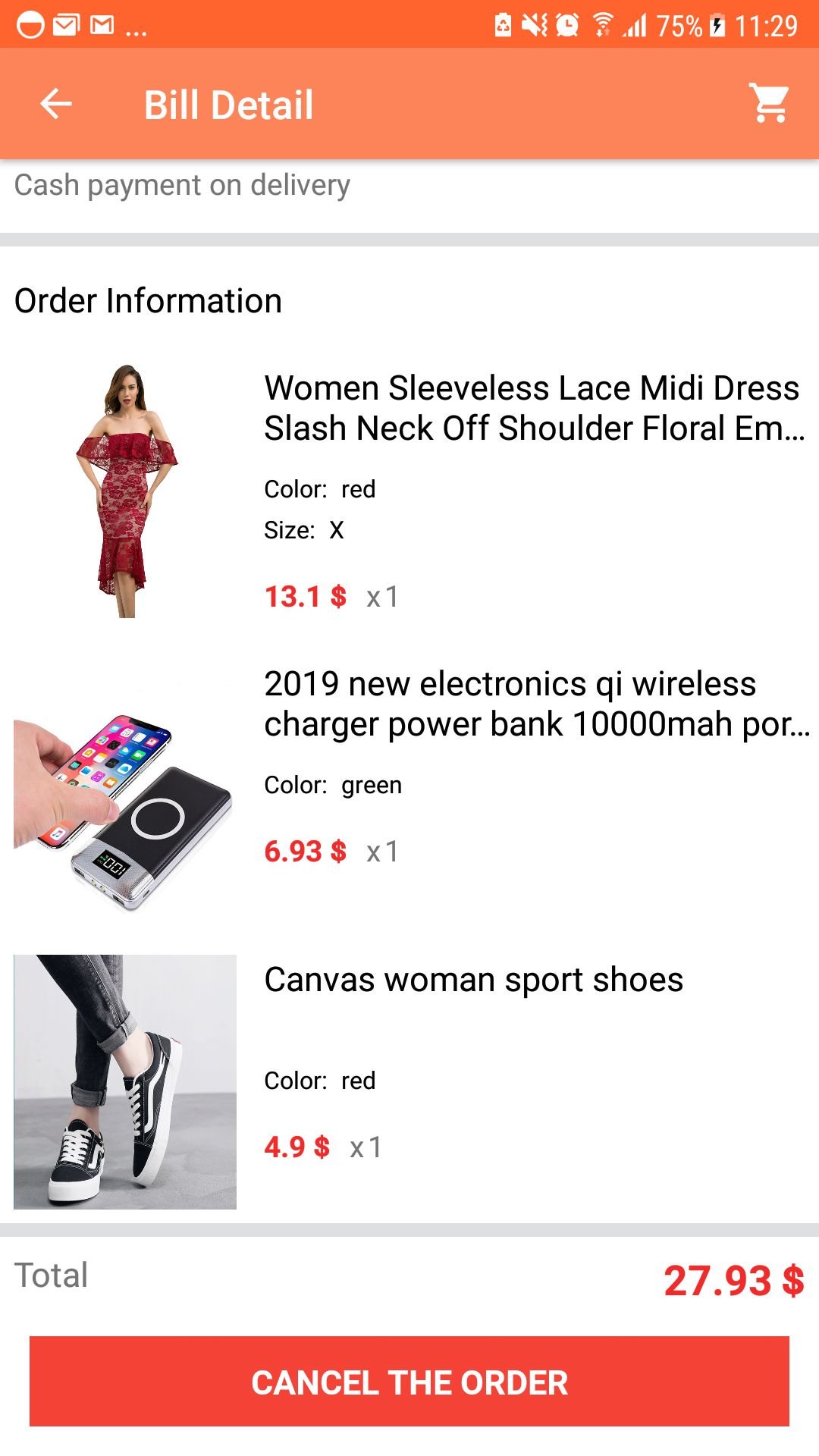This image is a screenshot of a mobile phone displaying a checkout page. The page is titled "Bill Detail" located at the top left-hand corner with a back arrow button beside it. The top right-hand corner features a white shopping cart icon, which likely redirects to the shopping cart view.

The checkout summary lists three items being purchased, each accompanied by a price and a thumbnail image: a woman's dress, a wireless charger power bank, and women's sports shoes. Detailed pricing information for these items is clearly provided next to their respective listings.

At the bottom of the screen, there's a prominently featured, large rectangular button with the text "Cancel Order" in the center. This button is displayed in a reddish-pink hue, making it easily noticeable. The total amount for the order is summarized as $27.93.

Overall, the page provides a comprehensive view of the order details, including individual item prices, pictures, and a clear option to cancel the order at the bottom.